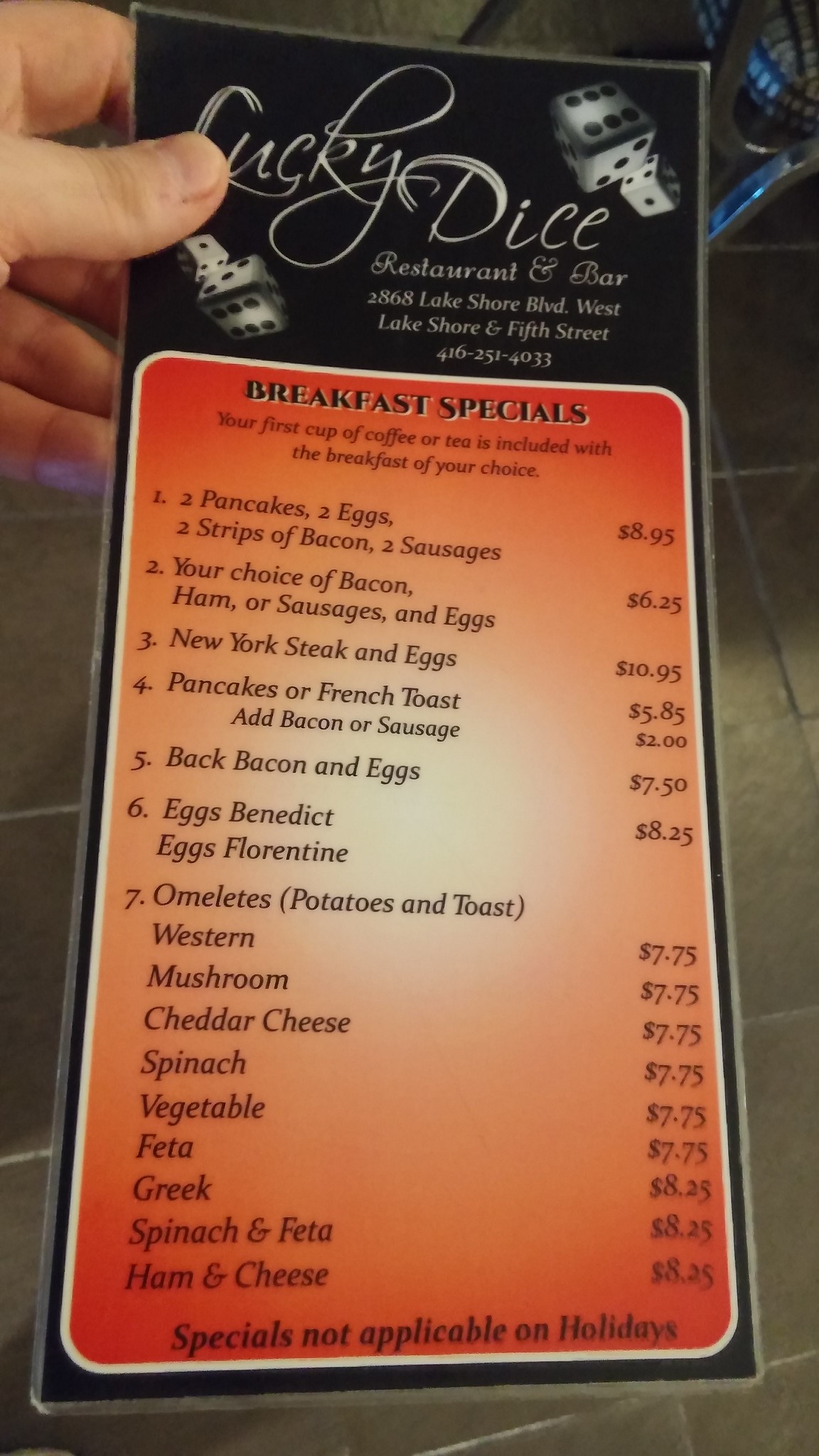The menu from Lucky Dice Restaurant and Bar, located at 2868 Lakeshore Blvd West on the corner of Lakeshore and 5th St (contact: 416-251-4033), features a black, laminated background with a sophisticated cursive-style "Lucky Dice" at the top. This title is accentuated with an illustration of two dice in the top right corner: the larger die shows a 6 on top and a 3 on the side, while the smaller die below it reveals a 3 on top and a 6 on the side, and another die shows a 1.

Below this, in the central area of the menu, you will find a list of breakfast specials. The first cup of coffee or tea is included with each breakfast choice. Offerings include:
- Breakfast Combo: 2 pancakes, 2 eggs, 2 strips of bacon, and 2 sausages for $8.95.
- Your choice of bacon, ham, or sausages with eggs for $6.25.
- New York steak and eggs for $10.95.
- Pancakes or French toast with the option to add bacon or sausage for an extra $2, priced at $5.95.
- Back bacon and eggs for $7.50.
- Eggs Benedict or Eggs Florentine for $8.25.

Omelet options come served with potatoes and toast:
- Western, Mushroom, Cheddar Cheese, Spinach, and Vegetable omelets each for $7.75.
- Feta, Greek, Spinach and Feta, and Ham and Cheese omelets each for $8.25.

Please note, breakfast specials are not available on holidays.

The image also shows a hand holding the menu with a black tiled background and a chair visible in the back right corner.